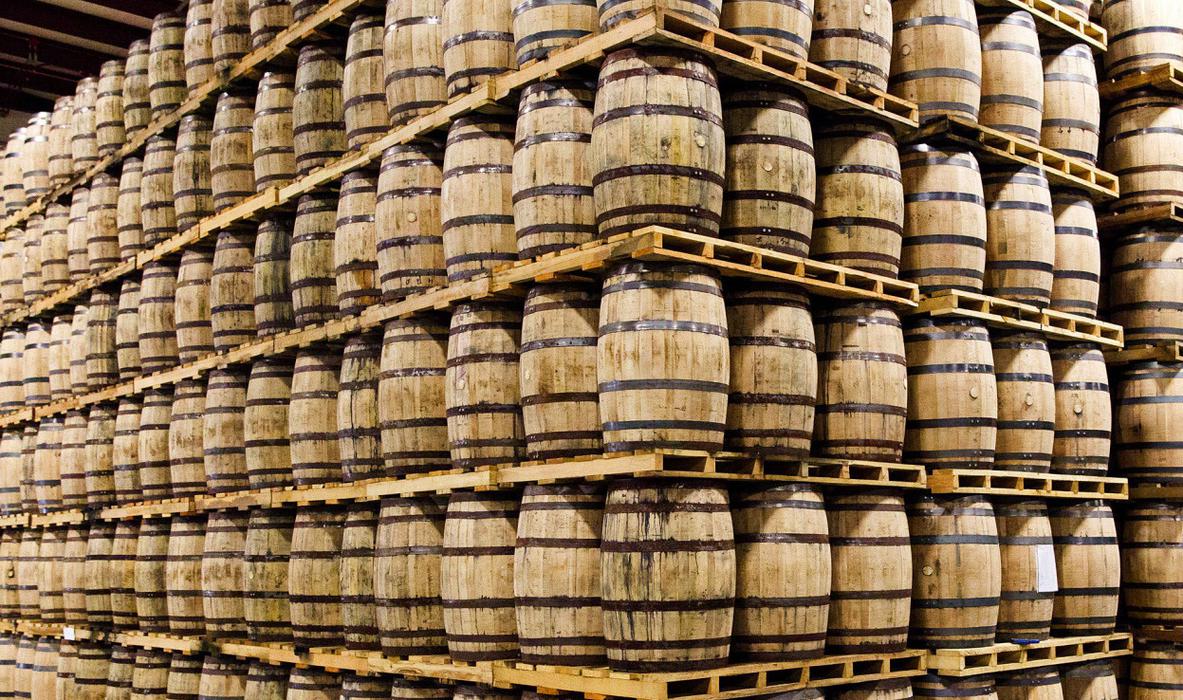The photograph depicts an extensive storage of wine barrels within a warehouse, meticulously organized into six towering rows of pallets, stretching upward to at least 20 feet. Each pallet row is interspersed with wooden boards, creating a stable structure that houses barrel after barrel, seemingly reaching the warehouse ceiling. The barrels, aged and weathered, are a light tan color, bound together by dark brown metal straps, with small dowel-plugged holes for access. Some barrels show red wine stains, adding character to their surfaces. Visible in the upper left corner of the image, the ceiling's open brown wood rafters hint at the warehouse's rustic construction. The entire right side of the image mirrors the left, emphasizing the vast quantity of wine barrels stored in this sprawling, orderly fashion.